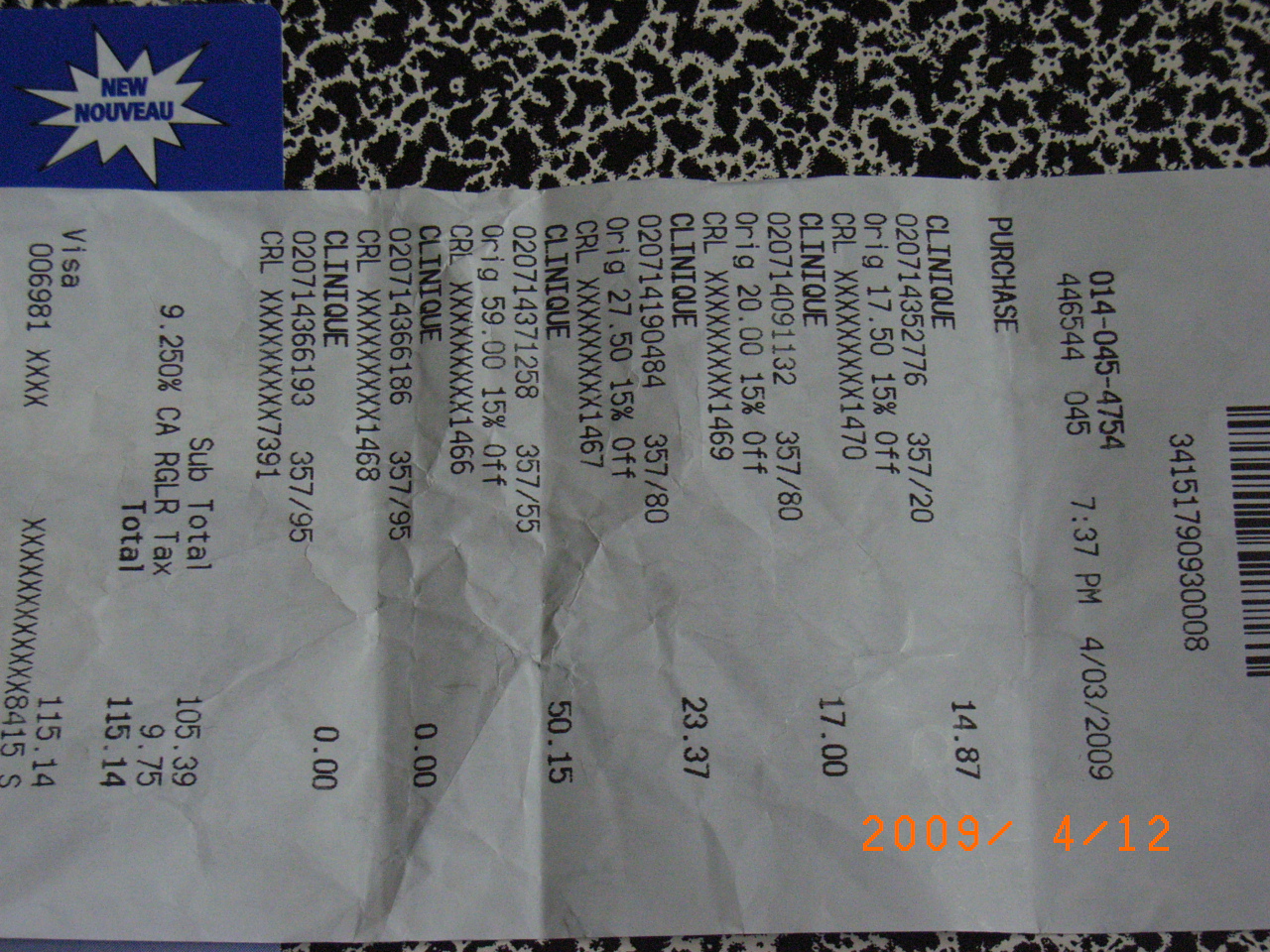A detailed photograph captures a receipt laid sideways against a backdrop. In the upper left corner of the image, a prominent blue square features a complex white star composed of numerous triangles, with the word "NUNOVU" displayed in blue lettering within the star. Adjacent to this, on the right, is a black rectangle adorned with an intricate pattern of white squiggly lines.

The receipt itself is white, with a vertically centered barcode on the right side, accompanied by a sequence of numbers directly below it. Following this, another set of numbers appears beneath the initial row. Towards the left side of the receipt, beneath these numbers, the word "Purchase" is clearly printed. Underneath this heading, a list of purchased items is detailed on the left side, each item paired with its respective price aligned on the right. The total amount for the purchases is positioned at the bottom of the receipt, completing the detailed transaction record.